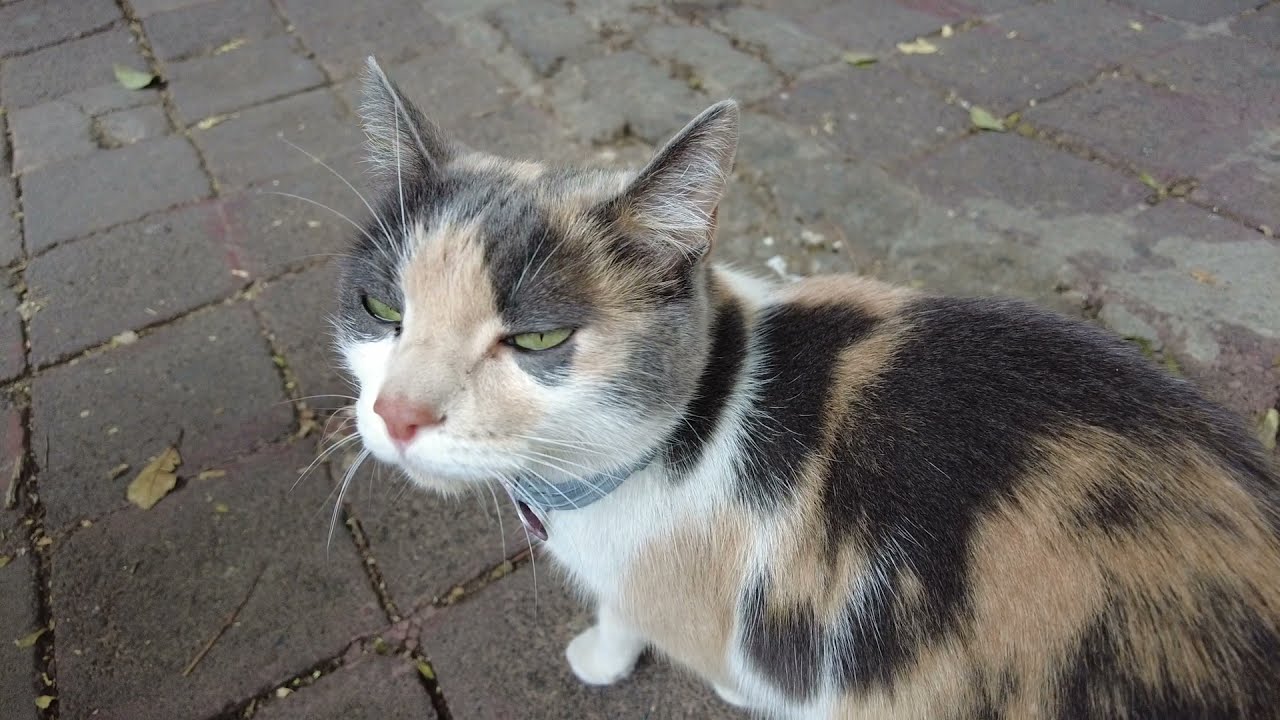This close-up image captures a calico cat, positioned on a craggy, mismatched brick-paved area with scattered leaves, suggesting the season might be fall. The cat, slightly scowling with mid-blink hazel green eyes, appears to be looking directly at the camera, giving it an almost intense expression. The feline sports a pink nose and a blue-gray collar adorned with a copper-colored tag. The calico's fur is a blend of white, tan, gray, jet black, and taupe, featuring three distinct large black areas. The cat's predominantly white chest contrasts with a mix of light brown and black on its head. Notably, the front left paw is entirely white, adding to its multicolored coat. The photograph captures nearly the entire body of the cat except for its tail and rear legs.